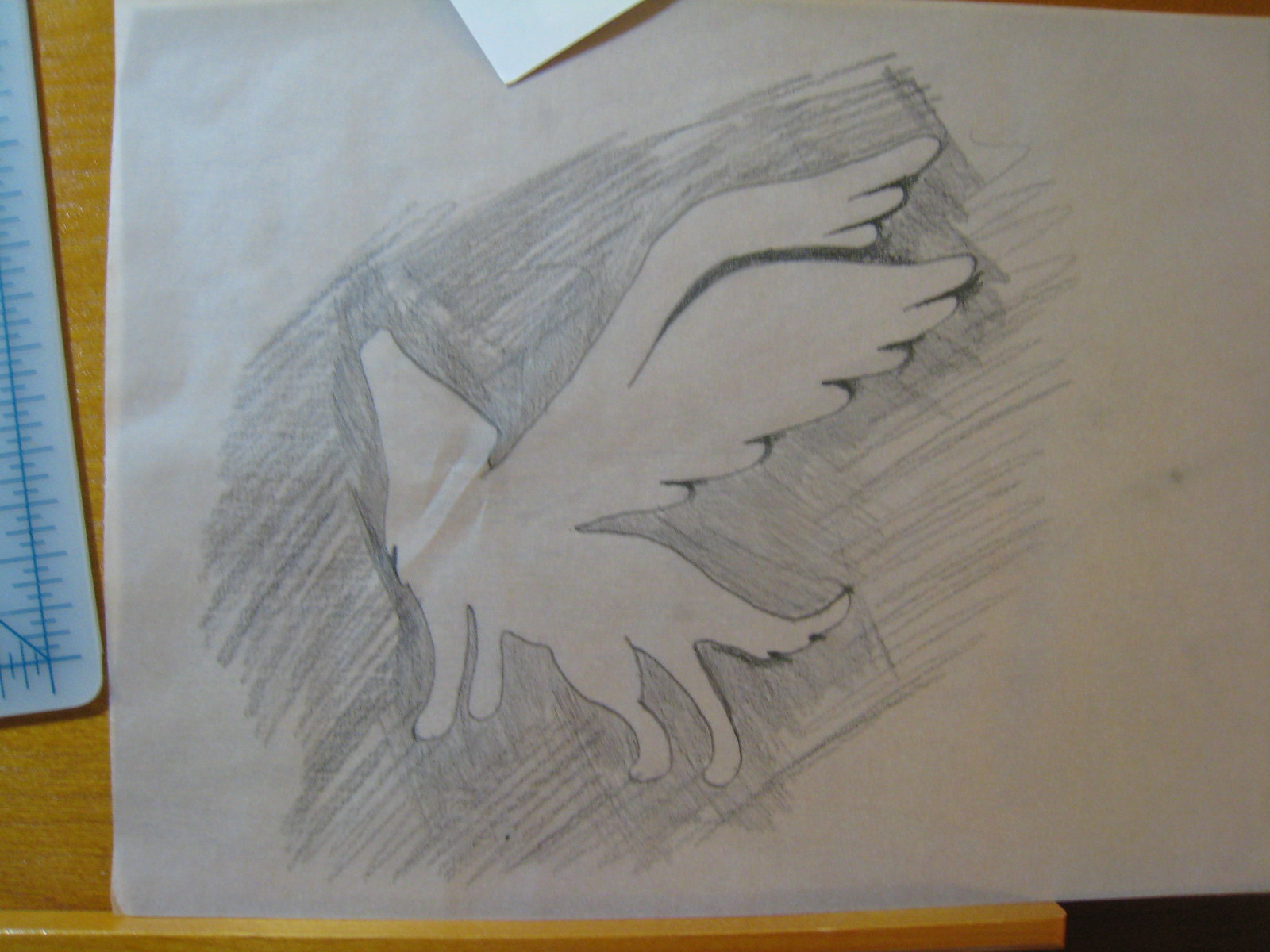This color photograph showcases a detailed pencil drawing on a plain white printer paper, laid out on a wooden surface. The artwork depicts the silhouette of a dog with a long, fluffy tail, standing on the ground with its head raised as if howling. The silhouette, entirely white, stands in contrast to the surrounding area, which has been shaded using the side of a graphite pencil. Distinctive to the drawing, a pair of large wings, darker at the edges, extends from the dog's shoulders, giving it an angelic, mythical appearance. To the left of the drawing, a blue and white ruler rests on the edge of the table, while the corner of another white piece of paper slightly overlaps the top center of the image. The paper holding the drawing extends past the wooden tabletop to the far right corner, adding a bit more depth to the composition.